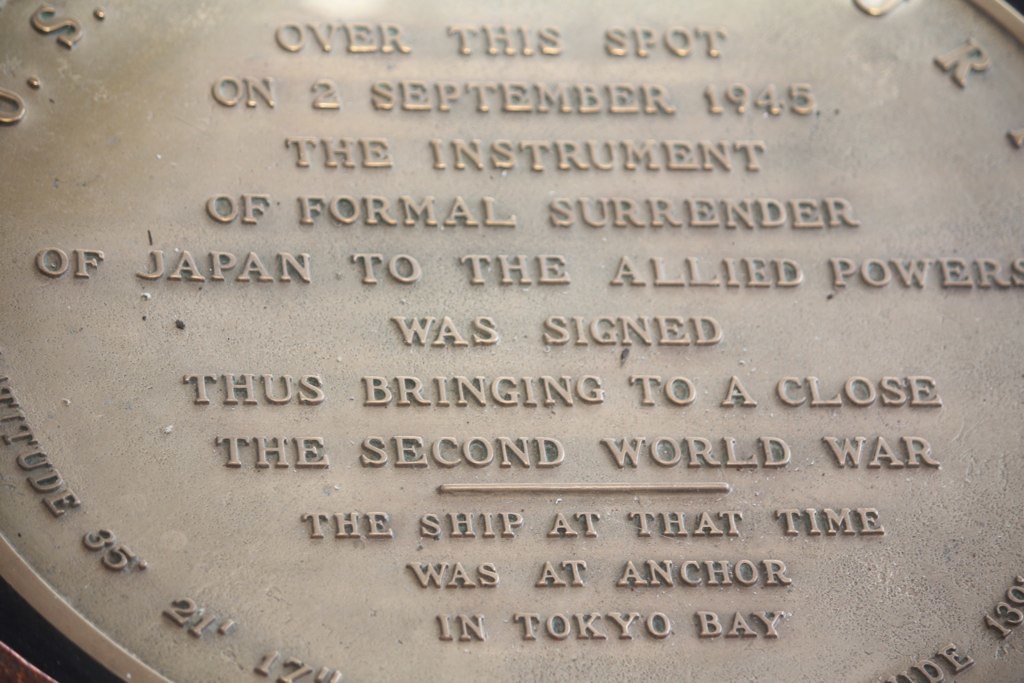This image captures a close-up of a large, circular metal plaque, likely made of bronze or iron, commemorating a significant historical event. The plaque, which resembles the size and shape of a sewer cover, is inscribed with a solemn message. It states that "Over this spot on September 2, 1945, the instrument of the formal surrender of Japan to the Allied powers was signed, thus bringing to a close the Second World War." This text is engraved prominently on the plaque. Below this, another inscription notes that "The ship at that time was at anchor in Tokyo Bay." The border of the plaque contains additional text, although some of it is obscured or cut off in the image, including phrases like "35 degrees attitude" and partial coordinates. The plaque serves as a memorial to the historic surrender ceremony that took place aboard the ship anchored in Tokyo Bay, marking the end of World War II.